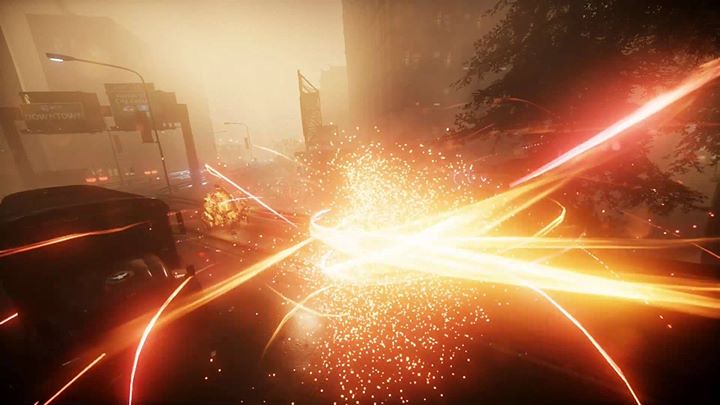This image is a night-time photograph of a cityscape featuring towering high rises in the background to the left and a highway stretching into the horizon. Highway signs with green backgrounds and white lettering, some displaying blue interstate symbols, are prominently suspended by massive columns over the roadway. Bent-over street lights project outward to illuminate the scene. The city's dark and murky ambiance is punctuated by a dazzling array of light swirls in the foreground. These swirls, resembling a thousand suspended sparkles or fireflies, display vibrant hues of yellow, red, and pink. The streams of light whirl around a central point, creating dynamic trails heading in multiple directions, including sideways, upward, and outward, almost like a mesmerizing shower of sparks. The juxtaposition of the bright, swirling lights against the cold, dark cityscape creates a striking visual contrast, making the light display the captivating focal point of the image.